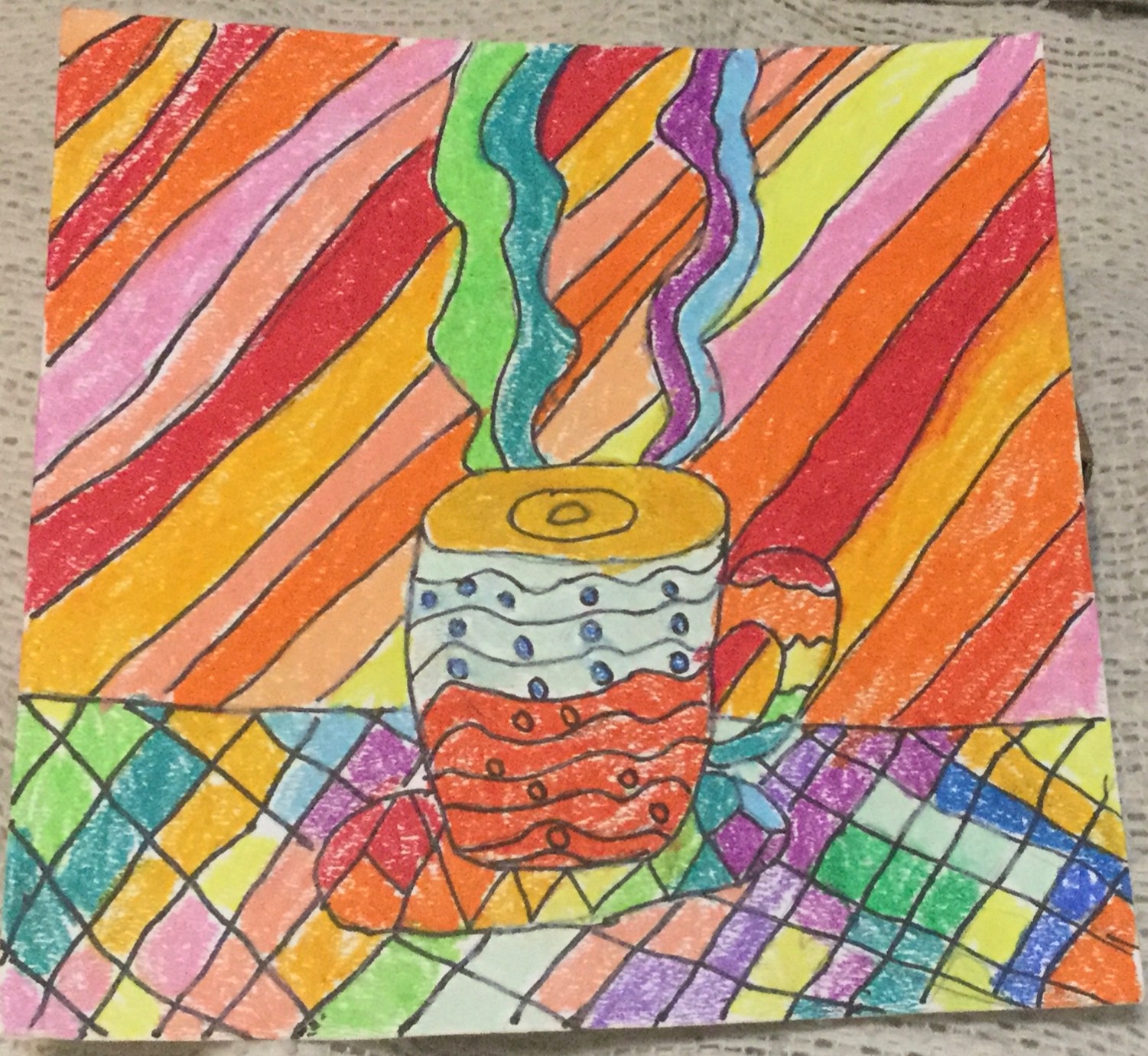This photograph captures a vibrant crayon drawing, placed on what appears to be a crocheted white doily, possibly outside on some sort of tarp, suggesting it might be up for sale. The artwork is dominated by a teacup resting on a saucer amidst an explosion of rainbow colors. The background features diagonally criss-crossing stripes in vivid hues of orange, red, yellow, purple, lavender, and green. At the bottom of the image, there is a checkerboard table design incorporating purple, blue, white, green, and yellow squares. The teacup itself is detailed with light blue and orange sections and adorned with blue and red wavy lines, complemented by circular dot patterns. Its handle displays a rainbow of colors. Rising from the cup, assumed to be filled with brown liquid, are trails of steam in shades of green, blue, purple, and light blue. The saucer beneath the cup mirrors the colorful theme with green, orange, red, and yellow zig-zag patterns.